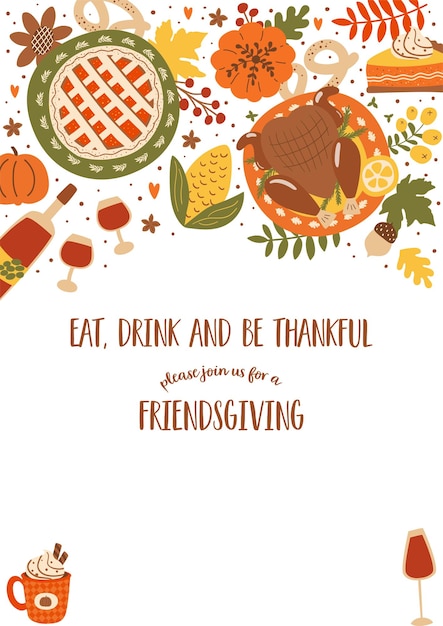This vertical, portrait-oriented Thanksgiving invitation features a festive, computer-generated collage occupying the top 40% of the image. The collage includes classic Thanksgiving symbols like a roasted brown turkey on an orange plate surrounded by flowers, ears of corn, whole pumpkins, and several pies, including a pumpkin pie and a lattice-topped fruit pie. There are also bottles of wine and wine glasses interspersed among the other elements. 

Centered just below this Thanksgiving spread, in brown text, the invitation reads, "Eat, Drink, and Be Thankful," followed by "Please join us for a Friendsgiving" in a mix of cursive and regular fonts. The lower part of the image showcases additional cozy details: a cup of hot cocoa with whipped cream and cinnamon sticks in the bottom left corner, and a glass of red wine in the bottom right corner. The overall design is both colorful and inviting, perfect for setting the tone for a festive Friendsgiving celebration.